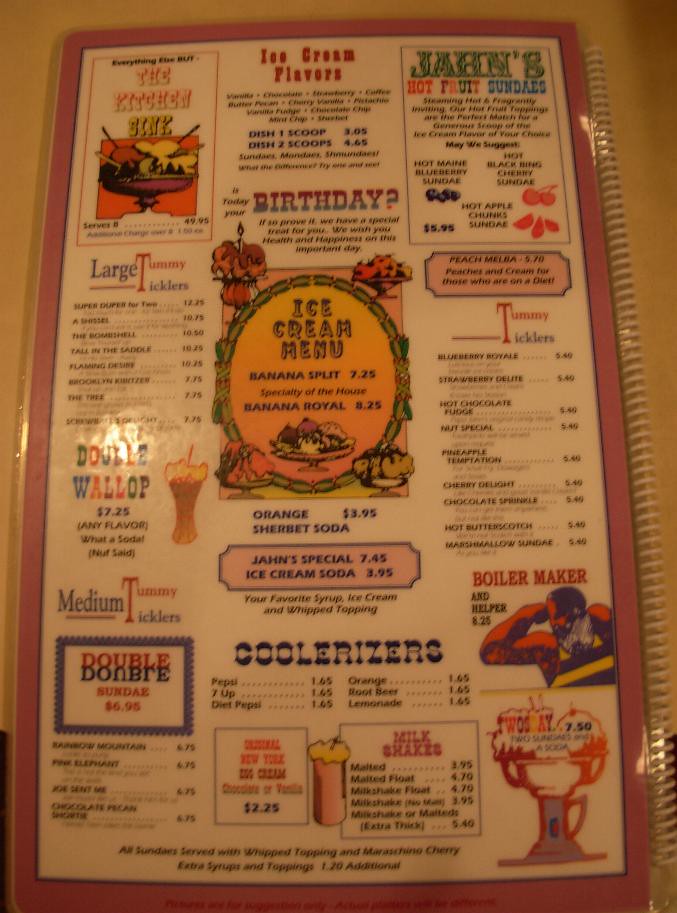The image captures an ice cream menu, seemingly from a restaurant, though it appears slightly blurry, making some items difficult to decipher. Dominating the central section are popular ice cream treats like Banana Splits and Banana Royals, prominently advertised to attract attention. Towards the lower part of the menu, a variety of drinks are listed, including Pepsi, 7-Up, Diet Pepsi, orange juice, root beer, and lemonade. The menu also showcases an array of delectable sundaes and milkshakes. On the right-hand side, several enticing dessert options are displayed, such as Hot Butterscotch, Marshmallow Sundae, Pineapple Temptation, Fruit Special, and Hot Chocolate Fudge. Scattered across the menu are small clip art illustrations of ice cream and milkshakes, adding a playful touch.